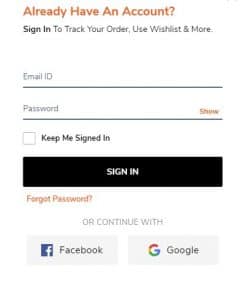This is a color portrait-oriented screenshot of a sign-in page from a website or app, viewed on a mobile device or possibly a computer. The interface prompts the user to enter their login details. At the top, it poses the question in orange text, "Already have an account?" followed by a black text instruction, "Sign in to track your order, use wish list, and more." Below this prompt are fields where users can input their email ID and password.

A "Keep me signed in" checkbox is available for users who prefer not to re-enter their login information each time. Once the fields are filled, the user can click a prominent black "Sign In" button.

Alternatively, users have the option to sign in through Facebook or Google by clicking on the corresponding icons, provided they are already logged into one of these platforms. The current screenshot shows that no user data has been entered in the fields yet. The image quality is slightly pixelated, making the text less sharp but still legible. The overall background is predominantly white.